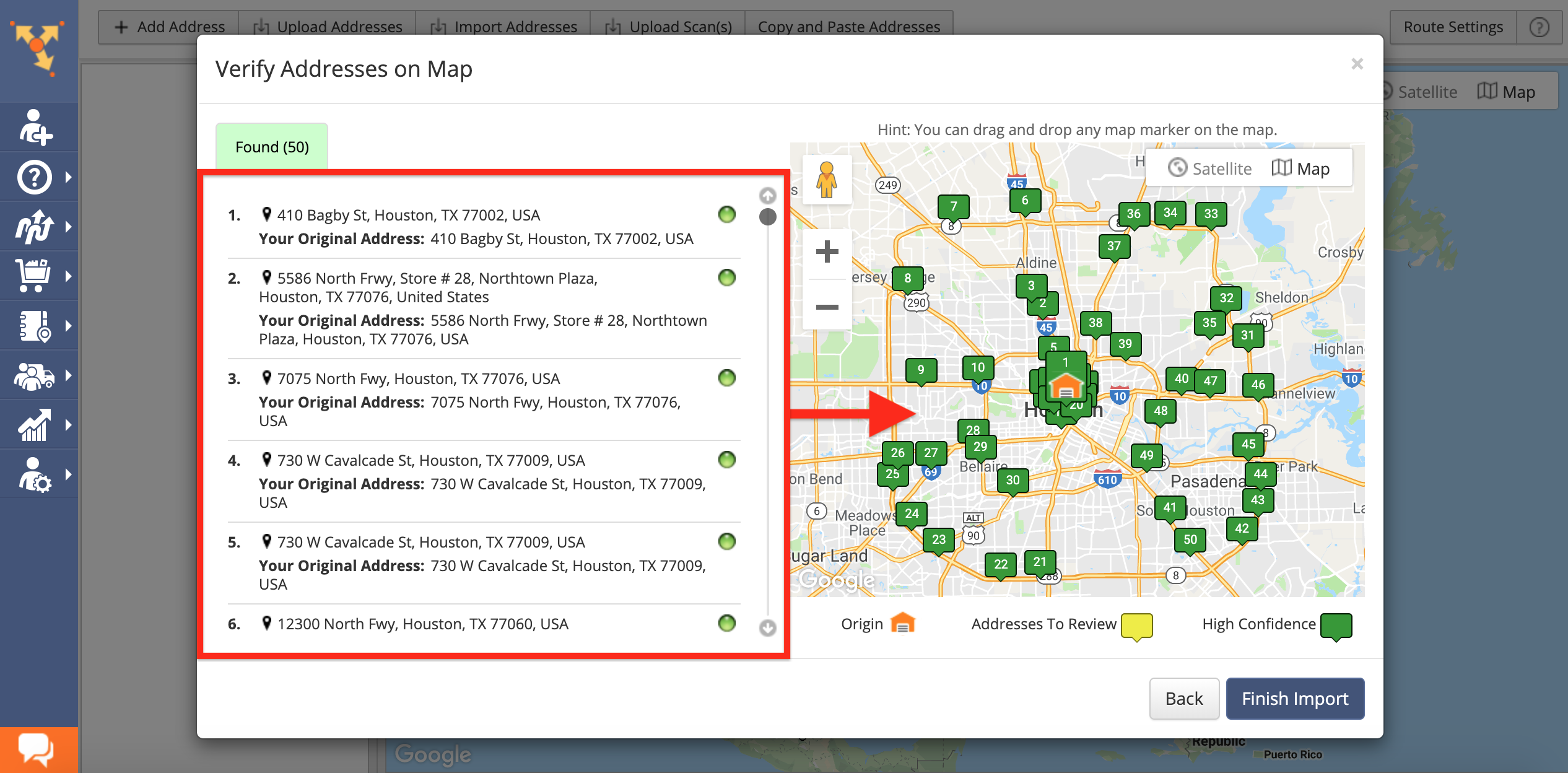The image showcases a detailed view of an application designed for map-related tasks, likely for verifying addresses. The central focus is the main workspace, a large map interface dominated by various icons, primarily green ones with numbers. The map is contained within a white box that is labeled "Verify addresses on map" at the top.

The interface includes a section labeled "Found" with a tally of '50', indicating the number of addresses found. Displayed below this label are the first six entries, with the capability to scroll through all 50 entries. An example of an address listed is "410 Bagby Street, Houston, Texas, 77002, USA."

On the right side of the main screen, the map plots several locations, possibly not all 50, with an icon legend nearby. The legend indicates:
- Origin point (icon design not specified)
- Addresses to review (yellow icon)
- High confidence addresses (green icon)

In the background, another map is visible, along with an assortment of icons at the top for functions such as "Add Address," "Upload Addresses," "Import Addresses," "Upload Scans," and "Copy and Paste Address."

To the left side of the interface is a blue navigation pane featuring multiple clickable icons for various site functions. At the bottom of this pane is an orange check bar or chat button, seemingly for user support.

The overall layout suggests a robust and multi-functional application focused on address validation and mapping, with tools for adding, uploading, and managing addresses efficiently.